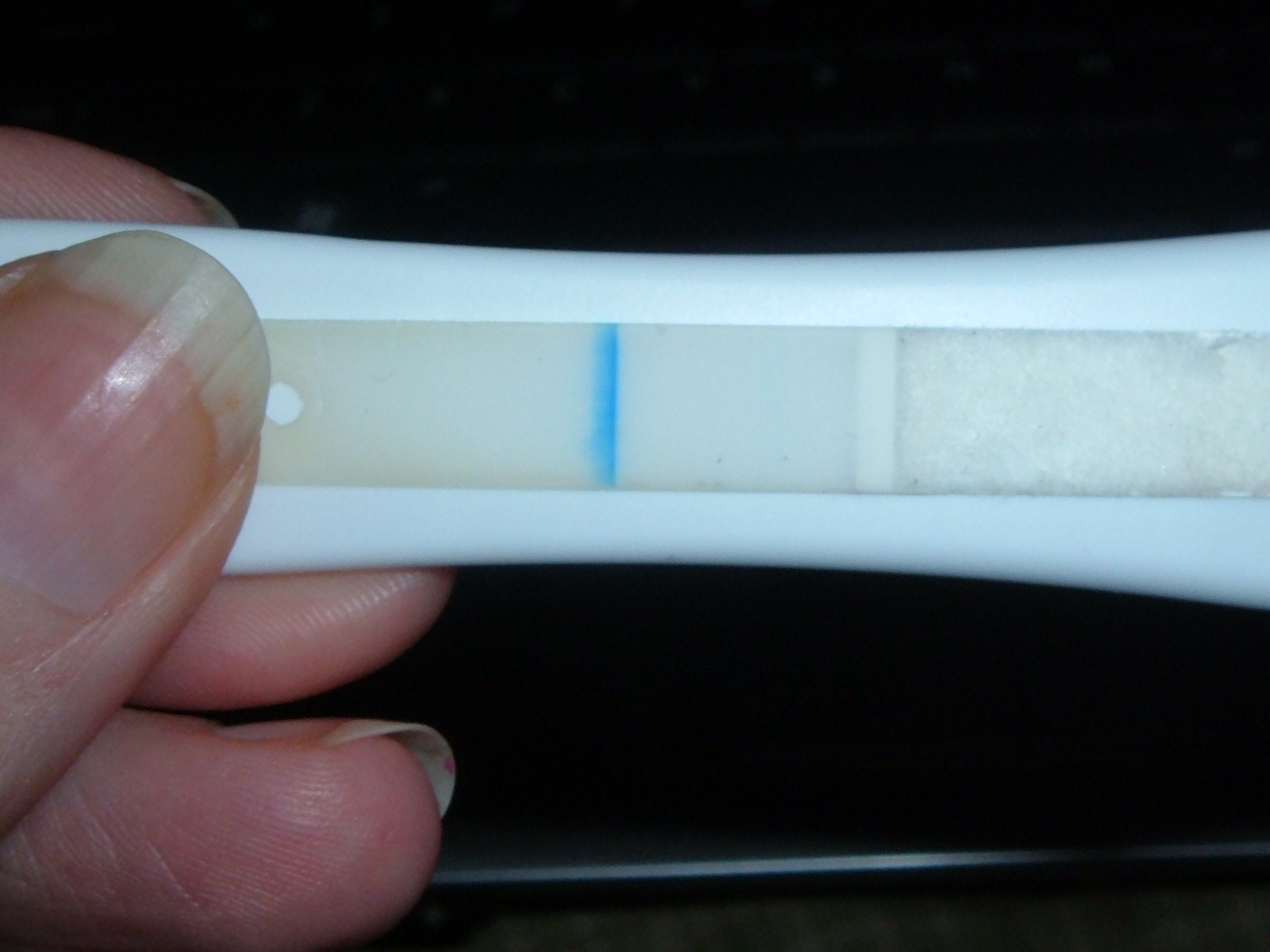In this close-up photograph, captured with a regular camera, the image is zoomed in to show the tips of a person's fingers and fingernails in astonishing detail. The person's fingerprints and the intricate wrinkles in their skin are clearly visible due to the extreme zoom. The background is a deep black, adding stark contrast to the scene, with a subtle reflection of light running horizontally along the bottom.

The fingers are delicately holding a plastic-lined object that resembles a pregnancy test. A distinct blue line is visible in the middle of the test, while the rest of the device appears predominantly white, though slightly dingy and grayish towards one end, giving it a somewhat worn appearance. A circular hole at one end of the object reveals a glimpse of white through it.

Additional details of the fingers include a few specks of dirt beneath the fingernails and a noticeable reddish line where the nail bed meets the free edge of the nails. The longer length of the fingernails suggests that the subject might be a woman. The overall composition highlights both the texture of the skin and the specific features of the held object, creating a detailed and candid snapshot.